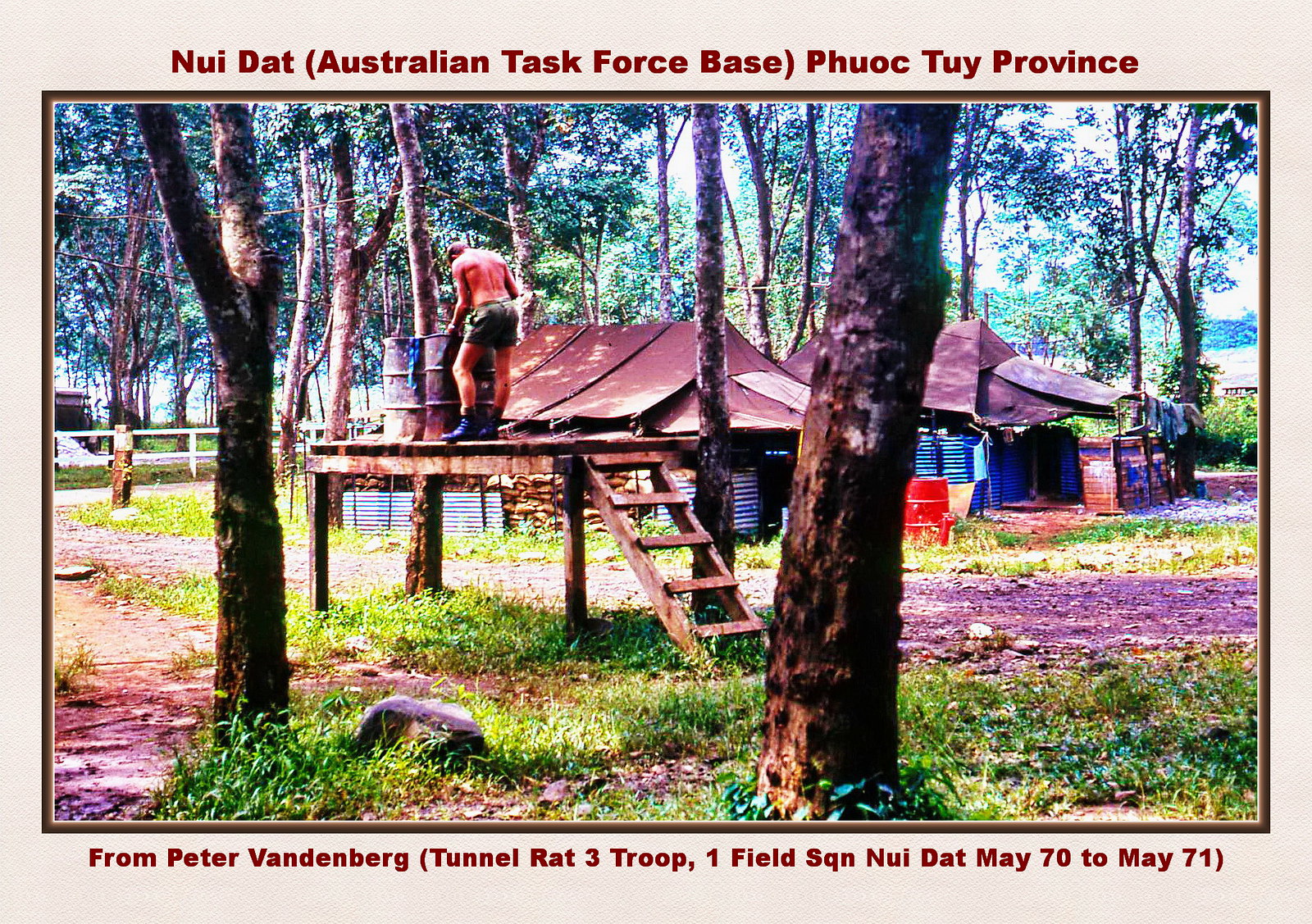This image captures a scene from the Australian Task Force Base in Phuoc Tuy Province, dated between May 1970 and May 1971, contributed by Peter Vandenberg of Tunnel Rat 3 Troop, One Field Squadron. Central to the image is a man with peach skin, dressed in green shorts and black boots, standing on a wooden platform. He is positioned slightly left of center and is engaged with two rusted, 50-gallon metal barrels in front of him. A wooden ladder with five boards ascends to the platform, which is attached between two deciduous trees with green foliage. The foreground showcases these trees with patches of grass and dirt.

Behind the man, the scene includes two makeshift tent-like structures, formed with tarps and wooden frames, sheltering blue objects and some chopped wood. Beyond these structures lies a more densely wooded area, with sunlight filtering through the leaves, illuminating parts of the clearing. The image features a mix of colors: green from the grass and trees, brown from the dirt and barrels, and blue from the objects under the tents. The photograph has a border with labels at the top and bottom, indicating its historical and military context.